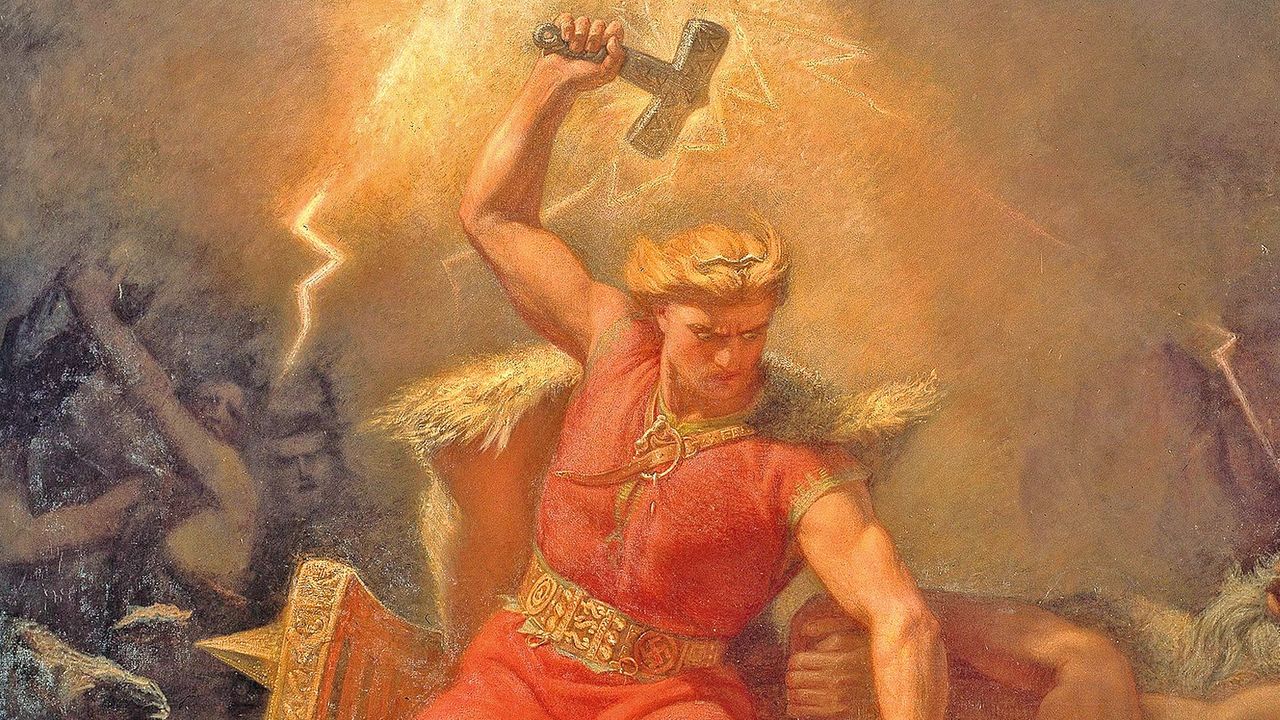This painting vividly captures the image of a powerful god-like man, reminiscent of Thor or Zeus. The central figure is a muscular, white man with blonde hair, who stands fiercely in the foreground. He wears a sleeveless red and orange garment cinched with a large gold belt, and a leather strap crosses his left shoulder holding up a fur cape that drapes behind him. His right hand is raised above his head, gripping a silver hammer from which lightning bolts descend, illuminating a yellow-orange background that fades to black towards the edges. The man appears to be looking down towards the right corner of the painting, preparing to bring the hammer down with immense force. The scene suggests impending chaos, heightened by the terrified expressions of the blurry figures to the left, who cling to each other in fear. Additionally, a bearded man lies at the bottom right corner of the image, further emphasizing the sense of turmoil and awe surrounding the central figure.